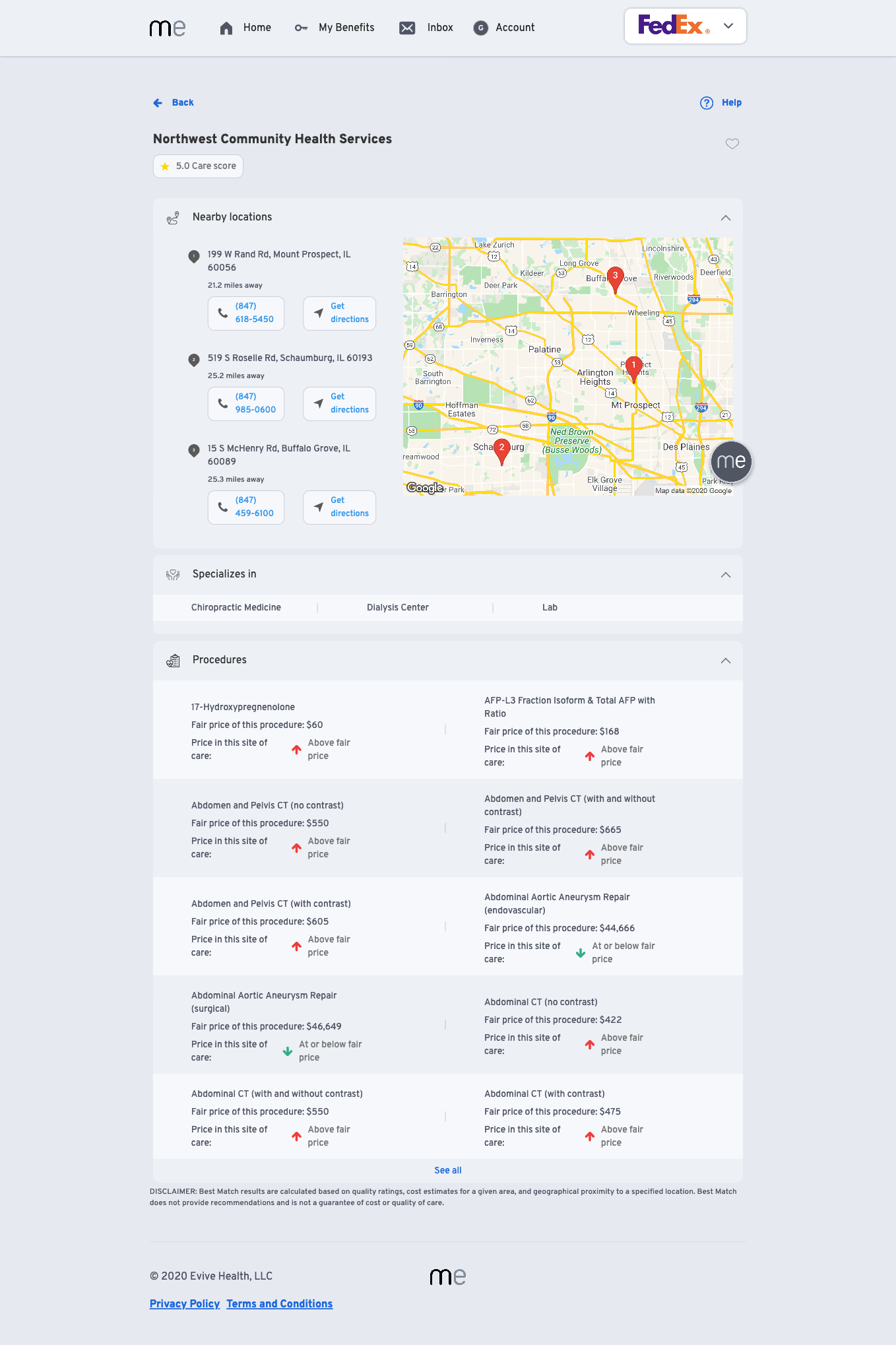Screenshot of a Tablet Displaying a Healthcare Website

The screenshot appears to be taken from a tablet, showing the navigation and content of a healthcare-related website. At the top, there are the letters "M" and "E," where "M" is in bold black font, and "E" is in a slightly lighter font. Below these letters, there is a standard navigation bar with icons and labels as follows:

1. **House Icon followed by "Home."**
2. **Key Icon followed by "My Benefits."**
3. **Envelope Icon followed by "Inbox."**
4. **Solid gray circle with a 'G' indicating Google followed by "Account."**

Next, the FedEx logo appears, with the familiar purple letters "FED" followed by an orange "X." Below this, there are options to go "Back" and access "Help," indicated by a question mark icon.

The main content area of the screenshot is focused on Northwest Community Health Services. The website displays a gold star icon with a "5.0 Care Score" next to it, indicating high-quality care.

Below this rating, the website lists the address "199 West Rand Road, Prospect, Illinois 60056" and provides a phone number for contact. Further down, there are listings for various hospitals and medical centers, each associated with a specific location.

A map is displayed, featuring red location tags marked 1, 2, and 3. These tags correspond to nearby healthcare facilities, specializing in chiropractic medicine, dialysis centers, and laboratory services. The map offers a visual representation of these locations, reflecting their geographic positions and available services.